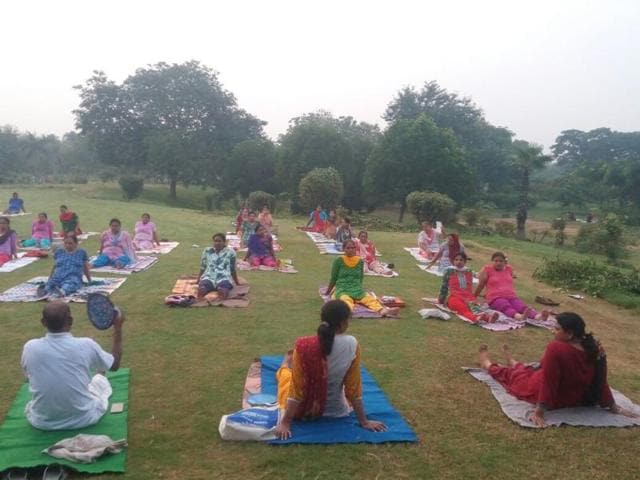The image depicts an outdoor gathering, possibly a yoga or meditation session, taking place in a vibrant, grassy park with scattered trees and shrubs. The sky appears semi-clear with intermittent clouds, and the atmosphere suggests a warm day, as some individuals are seen fanning themselves. The attendees, predominantly dressed in traditional Indian attire like bright saris and other colorful clothes, are seated on an array of multi-colored blankets, including shades of blue, green, white, and gray. They are arranged in approximately three rows; the front row is positioned with their backs to the camera, while the others face towards it. Central to the scene is a man in a white shirt, holding up an unknown object, capturing the attentive focus of the group. This vibrant and detailed scene is devoid of any additional text or objects, emphasizing the serene communal atmosphere.